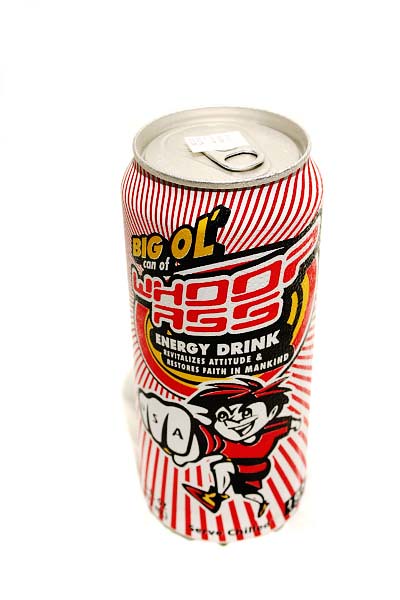Photograph of an energy drink can against a stark white background. The can is prominently displayed, with no other elements in the frame. The label features the bold, playful text "Big Ol' Can of Whoop Ass Energy Drink." The phrase "Big Ol'" is styled with an apostrophe replacing the 'd,' imparting a casual, irreverent tone. Below this, in smaller white letters, the can proudly claims to "Revitalize Attitude and Restore Faith in Mankind."

Adorning the can's busy, red-and-white-striped design is a lively illustration of a mischievous boy. He has spiky red hair, punches his fist out with his knuckles facing forward, and wears a red shirt that enhances his spirited appearance. The overall design is vibrant and eye-catching, reinforcing the playful and energetic branding of the product.